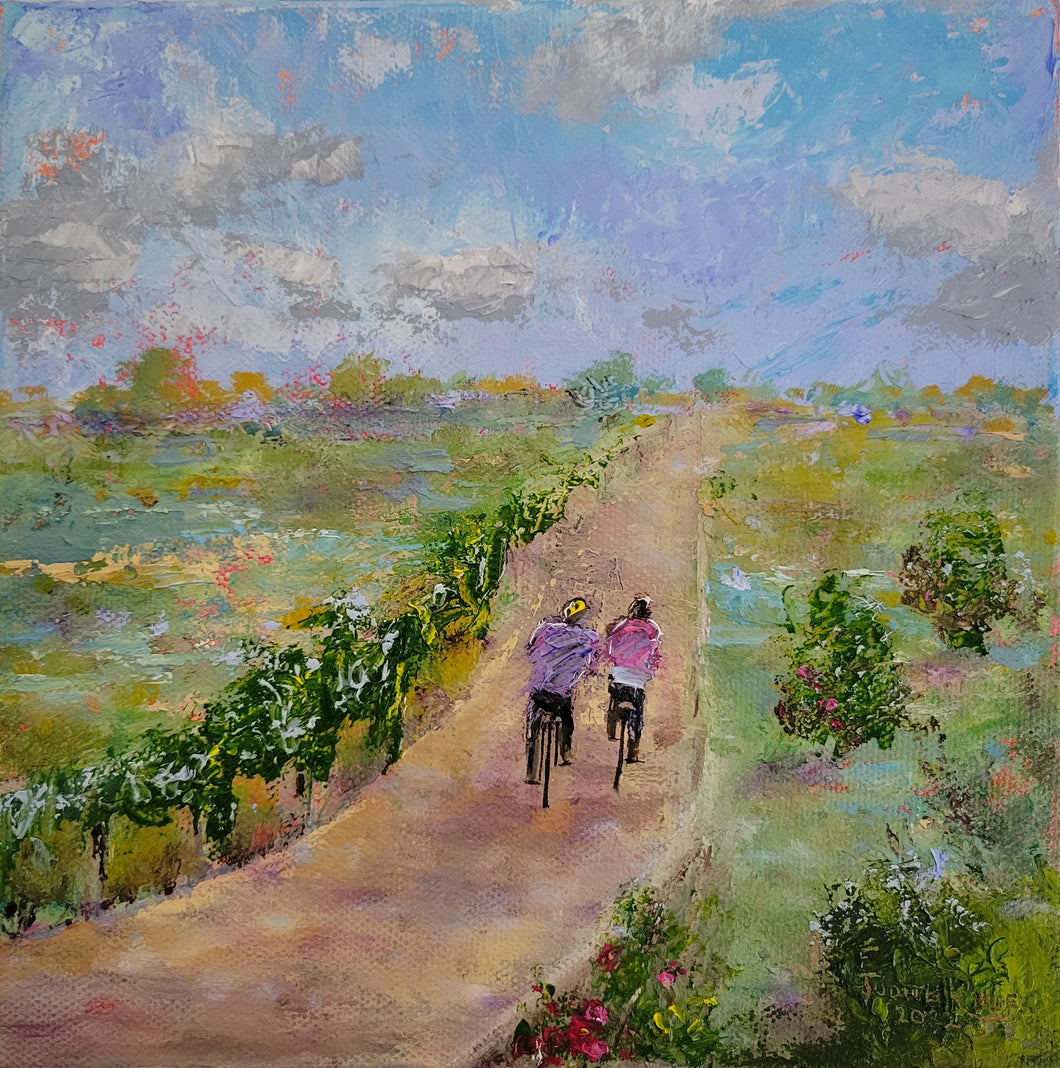This is a square oil painting on canvas that vividly depicts a serene landscape. Central to the painting is a winding dirt path of varying brown and pink hues, which curves from the bottom left horizontally and then vertically up to the middle right. On this path, two cyclists are riding their bikes: one in a purple top with a yellow helmet, positioned near the middle, and another in a pink top with a possibly black helmet. On the left side of the path lies a field adorned with low-lying vines or trees, stretching to the horizon. Additionally, several yellow and pink flowers, along with some shrubs, populate this grassy terrain. The horizon showcases a purplish-blue sky, accentuated with both white and dark gray clouds, suggesting a bright, sunny day. The entire scene is rich with green colors, enhancing the natural beauty of this outdoor setting as the cyclists appear to be heading towards a tranquil, picturesque expanse.